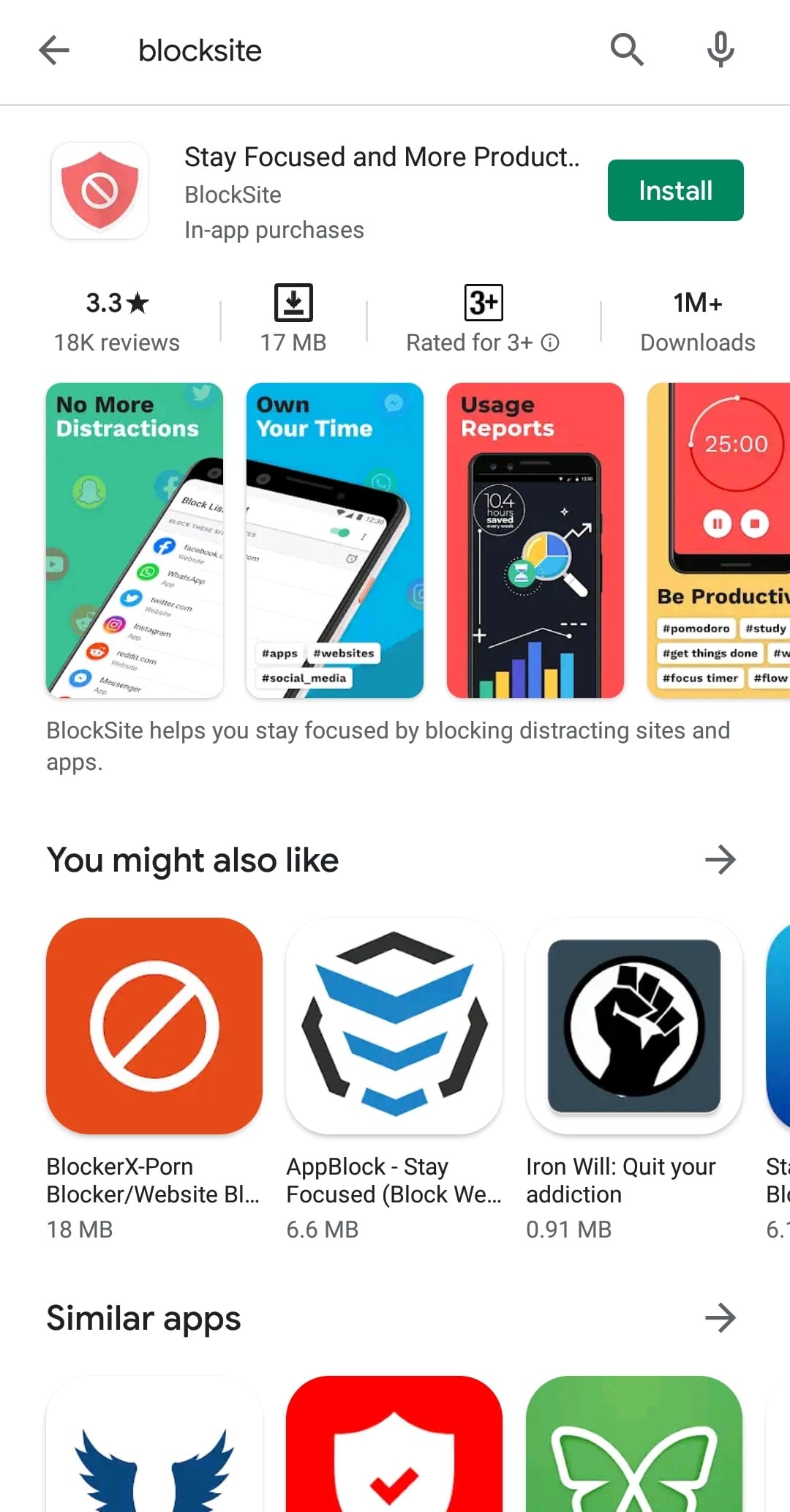This image depicts a screen from an app store. At the top, the screen title "Block Site" is prominently displayed within a search box. To the right of this title, there is a magnifying glass icon representing a search function and a speaker icon. On the left side of the title, there is a back arrow, indicating a navigation option to return to the previous screen.

Below the search box, the app name "Block Site" is highlighted again, together with its tagline "Stay Focused and More Productive." To the right of this information, there is a prominent green "Install" button. To provide additional context, the app has approximately 18,000 reviews, takes up a certain number of megabytes for download (exact size not mentioned), is rated for users ages three and up, and has been downloaded over 1 million times. The app's icon is also visible.

Further down the screen, a section titled "You Might Also Like" suggests other apps to the user. In this section, six different app icons and names are fully visible, showcasing alternatives related to blocking ads or managing digital habits.

The overall background of the screen is white, ensuring that the app details and suggestions are easily readable.